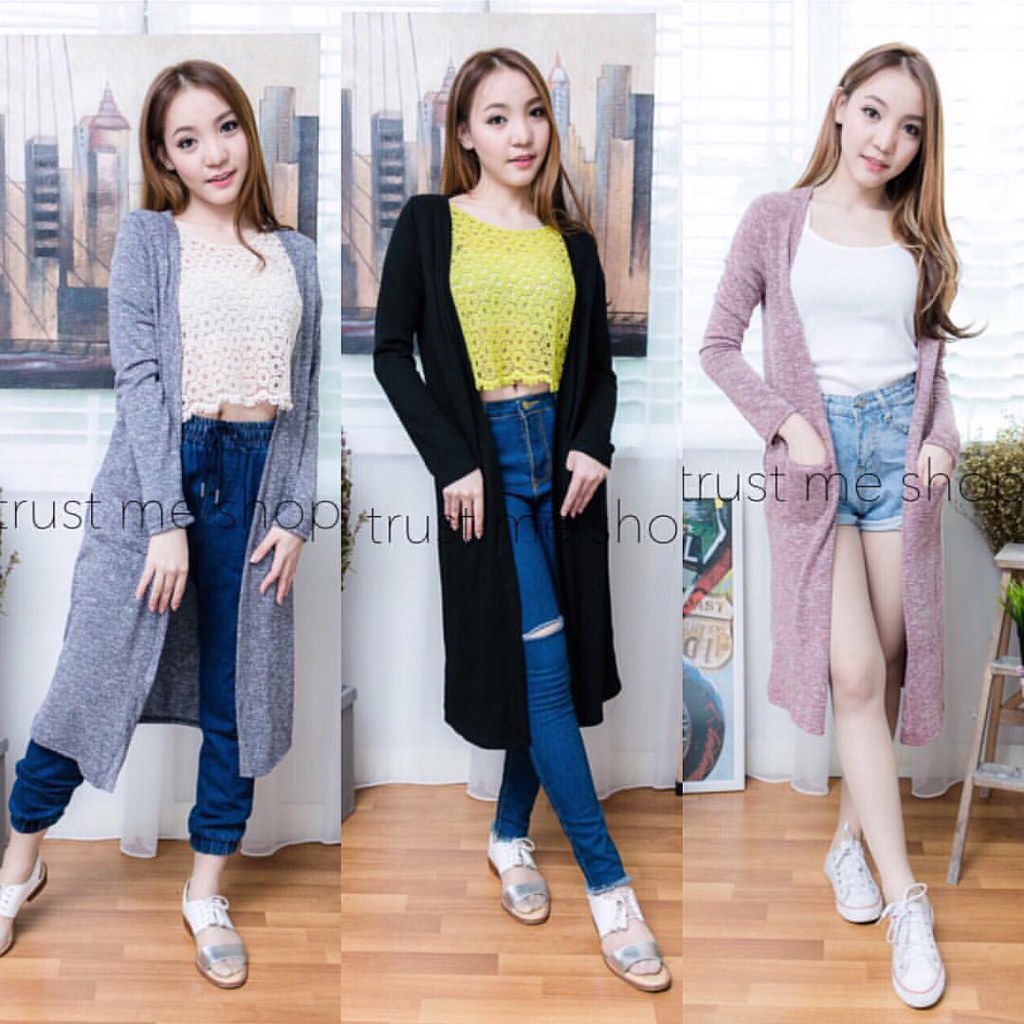This composite image features three vertical slices of the same pale-skinned Asian girl, each showing her in a different outfit. The leftmost slice depicts her in a long, light blue and white robe over a white mesh belly shirt, blue jeans, and sandals. In the center, she wears the same sandals, lighter blue jeans, a yellow mesh top, and a long black overcoat. The rightmost slice shows her in a long, light pink and white overcoat with short jean shorts, a white tank top, and white tennis shoes. The girl, standing on wooden flooring, has breast-length brown hair and is positioned in front of a window with closed white blinds. A cityscape painting is visible behind her in the first two slices, but absent in the third. Overlaid on the image in black text is the phrase "Trust Me Shop."